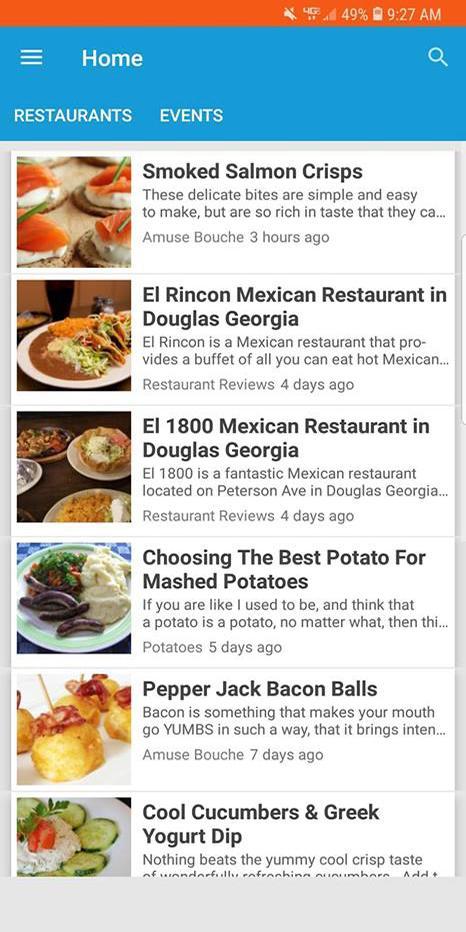The image depicts a mobile device screen characterized by its elongated rectangular shape. At the top, there's a dark orange status bar featuring several white symbols: a muted speaker icon indicating notifications or sound are off, '4G' for network status, a white signal strength indicator, '49%' showing the battery percentage, a battery icon, and the time '9:27 AM'.

Below the status bar, there's a medium blue navigation header. On the left, three white lines indicate a dropdown menu. Next to it, 'Home' is boldly displayed in white, followed by a white magnifying glass icon tilted to the left. 

Under this header, in capital lettering, are the sections 'RESTAURANTS' and 'EVENTS'. The main content begins with an image of four smoked salmon plates. The title "Smoked Salmon Crisps" is prominently displayed in black, bold font. Below this, a description reads, "These delicate bites are simple and easy to make, but are so rich in taste that they..." followed by an ellipsis. In light gray text, it states "amuse BOUCHE, three hours ago."

A thin gray divider line separates this from the next section, featuring an image of tacos. On the right, "El Rincon Mexican Restaurant in Douglas, Georgia" is written in black, bold letters. The description below notes, "El Rincon is a Mexican restaurant that pro-provides a buffet of all you can eat hot Mexican…" ending with an ellipsis. This is followed by "restaurant reviews, four days ago" in light gray text.

Further below, another image shows four different plates, accompanied by the title "L-1800 Mexican Restaurant in Douglas, Georgia" in black, bold lettering.